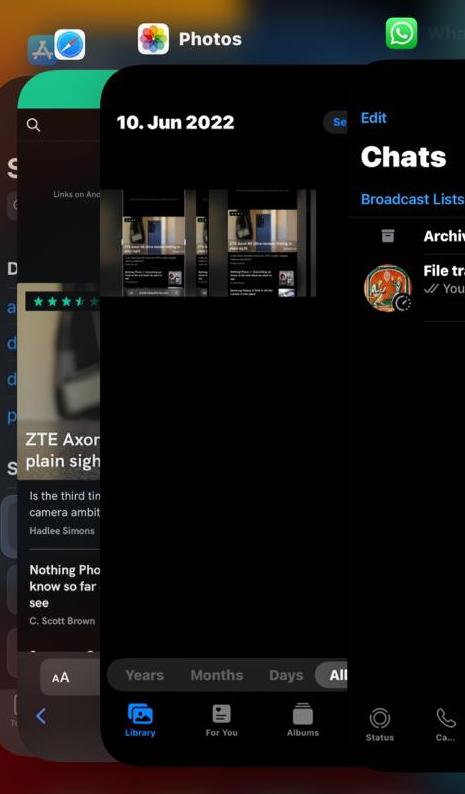The image is a vertically-oriented rectangular screenshot from a cell phone, showcasing multiple overlapping windows, partially obscured by each other. In the background, the phone's home screen is visible, with icons such as Photos, WhatsApp, and Compass lining the top and bottom of the screen. The primary open window on the left side displays fragments of text, including "zte8xor" and "plain sight," followed by the beginnings of what appear to be story titles: "is the third time camera let's see Hadley Simmons" and "nothing something see Scott Brown."

Overlapping this, another window is visible with the date "10th of June 2022" at the top. To the right of this window, options for "Chats," "Broadcast Lists," "Archives," and "File" are partially discernible. At the very bottom of this window, icons for "Library," "For You," "Albums," "Status," and "Call" are also evident. The screenshot captures the busy nature of multitasking on a smartphone, with layers of information and app interfaces vying for attention.